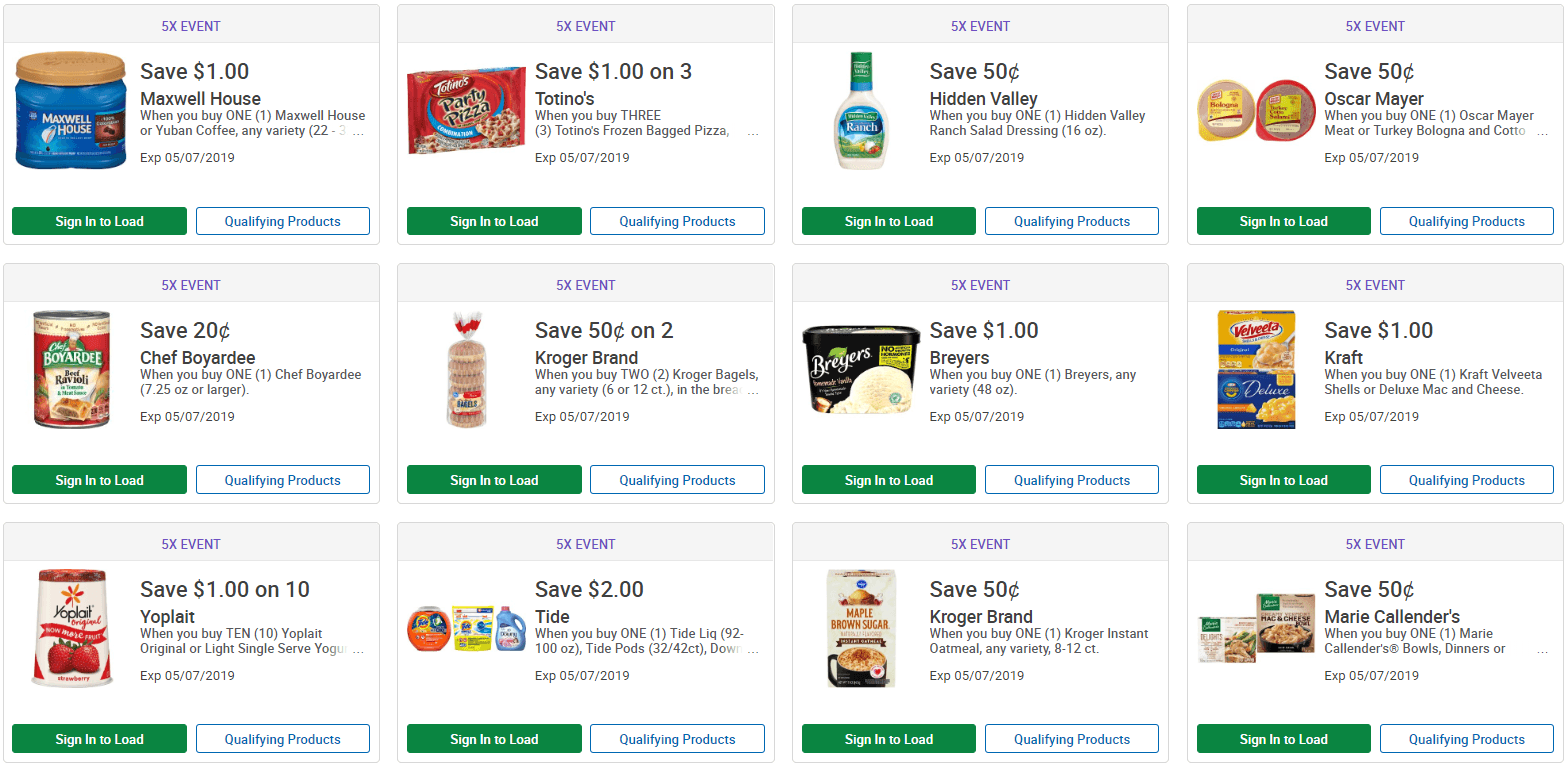This image displays a series of discount listings for various food items, prominently featuring notable brands and their respective savings offers. The items are detailed as follows:

1. **Maxwell House or Yuban Coffee**: Save $1 when you purchase any variety of Maxwell House or Yuban coffee.
2. **Totino's Products**: Save $1 when you buy three Totino's items.
3. **Hidden Valley Ranch Salad Dressing**: Save $0.50 when you buy one Hidden Valley Ranch Salad Dressing.
4. **Oscar Mayer Bologna**: Save $0.50 when you purchase one package of Oscar Mayer Bologna.
5. **Chef Boyardee**: Save $0.20 when you buy one Chef Boyardee product.
6. **Kroger Brand Bagels**: Save $0.50 when you buy two packs of Kroger Brand Bagels.
   
These promotions offer various savings on popular food items, making it an appealing assortment for budget-conscious shoppers.